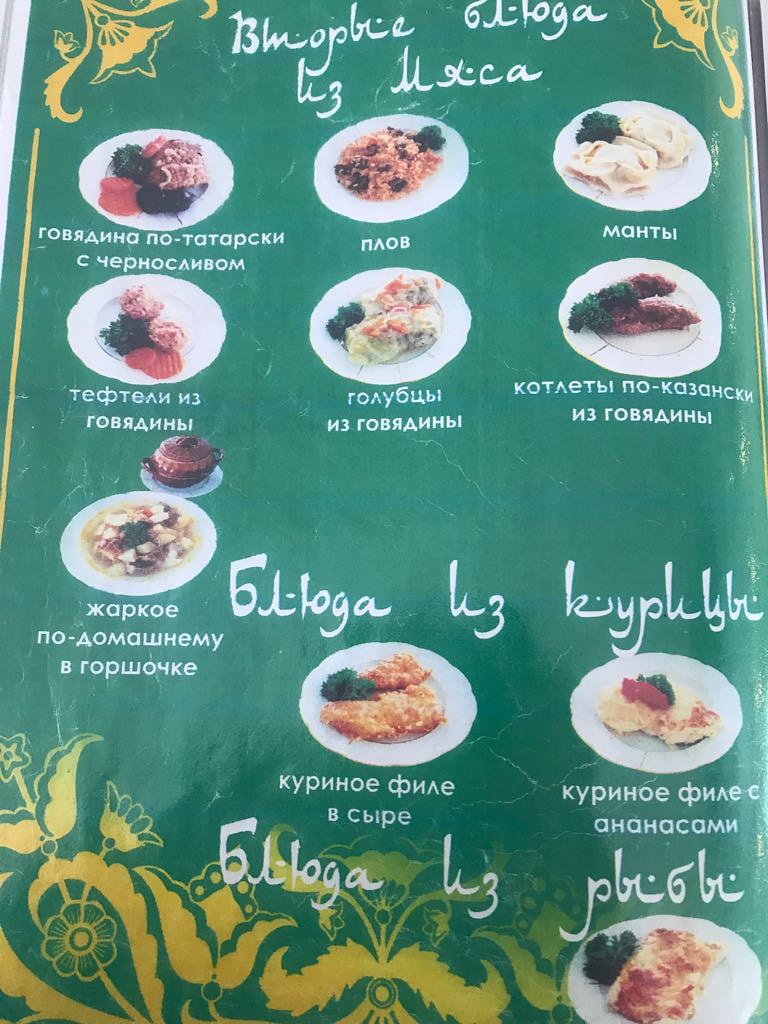The photograph features a vibrant food menu with a predominantly green background, embellished with intricate yellow floral designs in the top right and top left corners, as well as a matching yellow border. Additional floral decorations are present at the bottom of the menu, enhancing its aesthetic appeal. The menu itself displays a variety of dishes, arranged in a neat grid pattern.

The top section of the menu showcases six dishes, each presented on a white plate with a white background. These dishes are garnished with fresh green herbs and appear to contain rice, accompanied by either tomatoes or carrots as additional decorative elements. 

Moving to the bottom left of the menu, there's a dish that seems to feature potatoes in a soup, accompanied by a brown serving pot, adding a touch of rustic charm to the presentation.

Below this, under a specific heading, are two more dishes. The first is a serving of fried fish topped with green garnish, while the second resembles an omelette or pancake, also garnished with fresh herbs, maintaining a consistent theme throughout the menu.

Finally, in the extreme bottom right of the menu, there is a dish of baked potatoes, again garnished with green herbs, emphasizing a harmonious and visually appealing presentation. The text descriptions beneath each dish are written in a non-English language, adding to the authenticity and cultural richness of the menu.